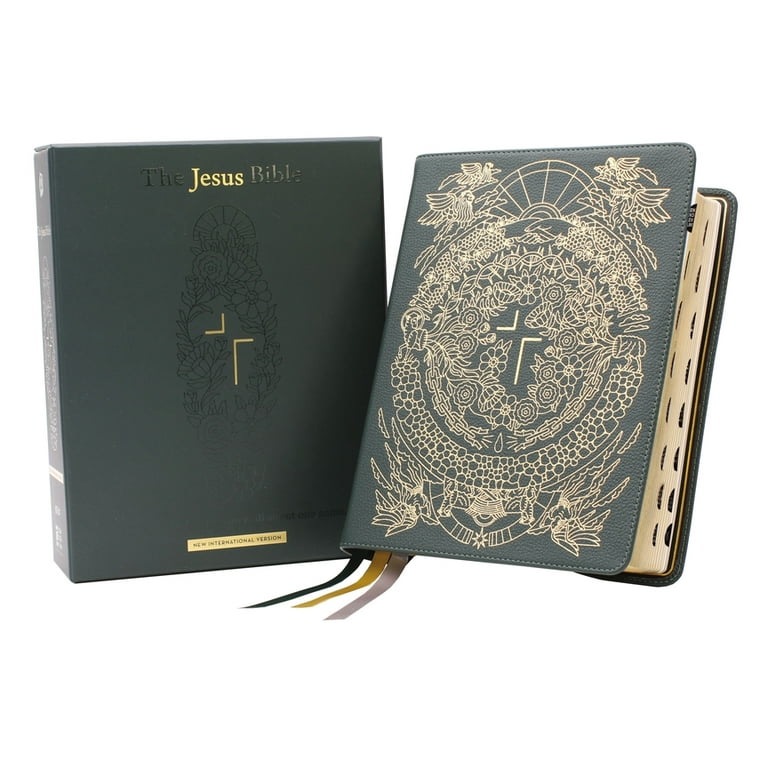This color photograph captures an ornate Bible and its accompanying storage box, with both items positioned at a slight diagonal. On the left is the storage box, dark green with a gold banner at the bottom that reads "New International Version" amidst hard-to-read small text and decorations. The box is titled "The Jesus Bible" with 'Jesus' written in gold and 'The' and 'Bible' in black, and it features an embossed floral design.

On the right is a highly detailed Bible with a dark green leather cover. The cover is adorned with gold embossed illustrations, including a symbolic cross surrounded by flowers, birds, and angels. The intricate design includes elements such as a sun, clasped hands, circles made of thorns and flowers, and a broken chain with a teardrop shape in the middle. The edges of the Bible reveal black tabs for easy navigation through different sections, while gold trim graces the interior around the pages. The Bible also features three satin bookmarks emerging from the bottom: one is black, another is yellow (or possibly orange), and the third is pale pink (or white).